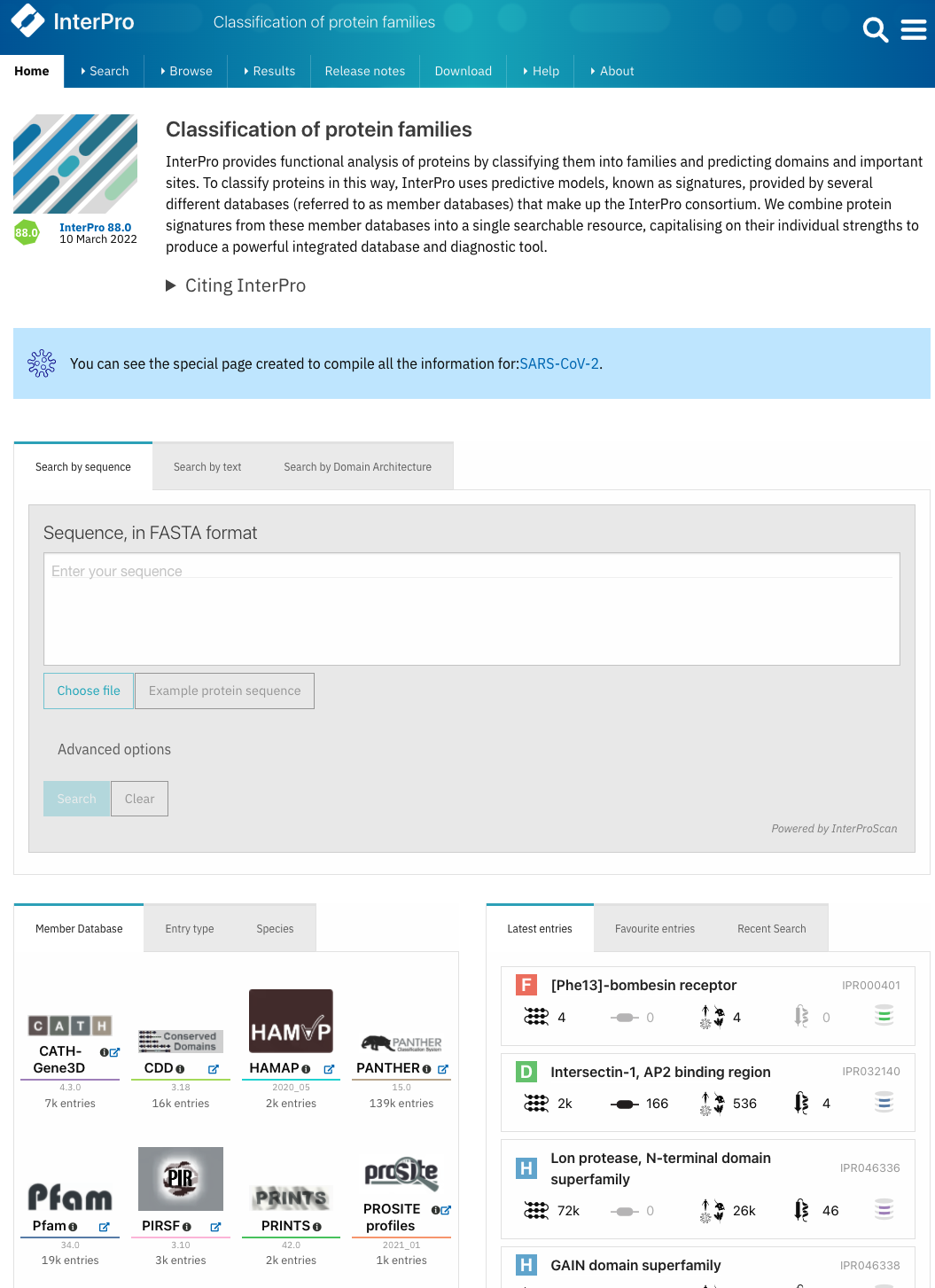This screenshot showcases the InterPro online interface, a bioinformatics resource dedicated to the classification of protein families. The interface is neatly split into several sections, with the "Home" section prominently highlighted. At the very top right corner, familiar symbols such as a magnifying glass for search functionality and a hamburger icon for additional options are visible.

A light blue rectangular banner extensively describes a special page created to provide comprehensive interaction information specifically for SARS-CoV-2 and SARS. Just below this banner, a box featuring sequences in FASTA format (with FASTA fully capitalized) is displayed, further facilitating detailed protein analysis.